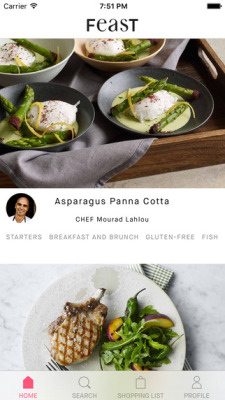The image showcases a mobile or tablet interface, featuring a culinary-themed screen. In the top left corner, "Carrier Centered" is displayed in black font, while the top right corner shows the time as 7:51 PM and the battery status icon. Centrally, a whimsical and playful font spells out "Feast." Below this header text, the following items are listed: "Asparagus Panna Cotta," "Chef Murad Lahou," "Starters Breakfast and Brunch," and "Gluten-Free Fish."

At the bottom of the screen, navigation icons for "Home," "Search," "Shopping List," and "Profile" are aligned horizontally. 

The main image features a wooden tray holding two artistic servings. Each serving includes a tortilla shell, garnished with cheese and sprinkled with bacon bits, accompanied by three pieces of asparagus topped with shredded cheese. Positioned behind this tray, another bowl holds a similar dish. Below the tray, a white plate showcases what appears to be either a grilled piece of chicken or fish, garnished with a variety of green vegetables artfully arranged around it.